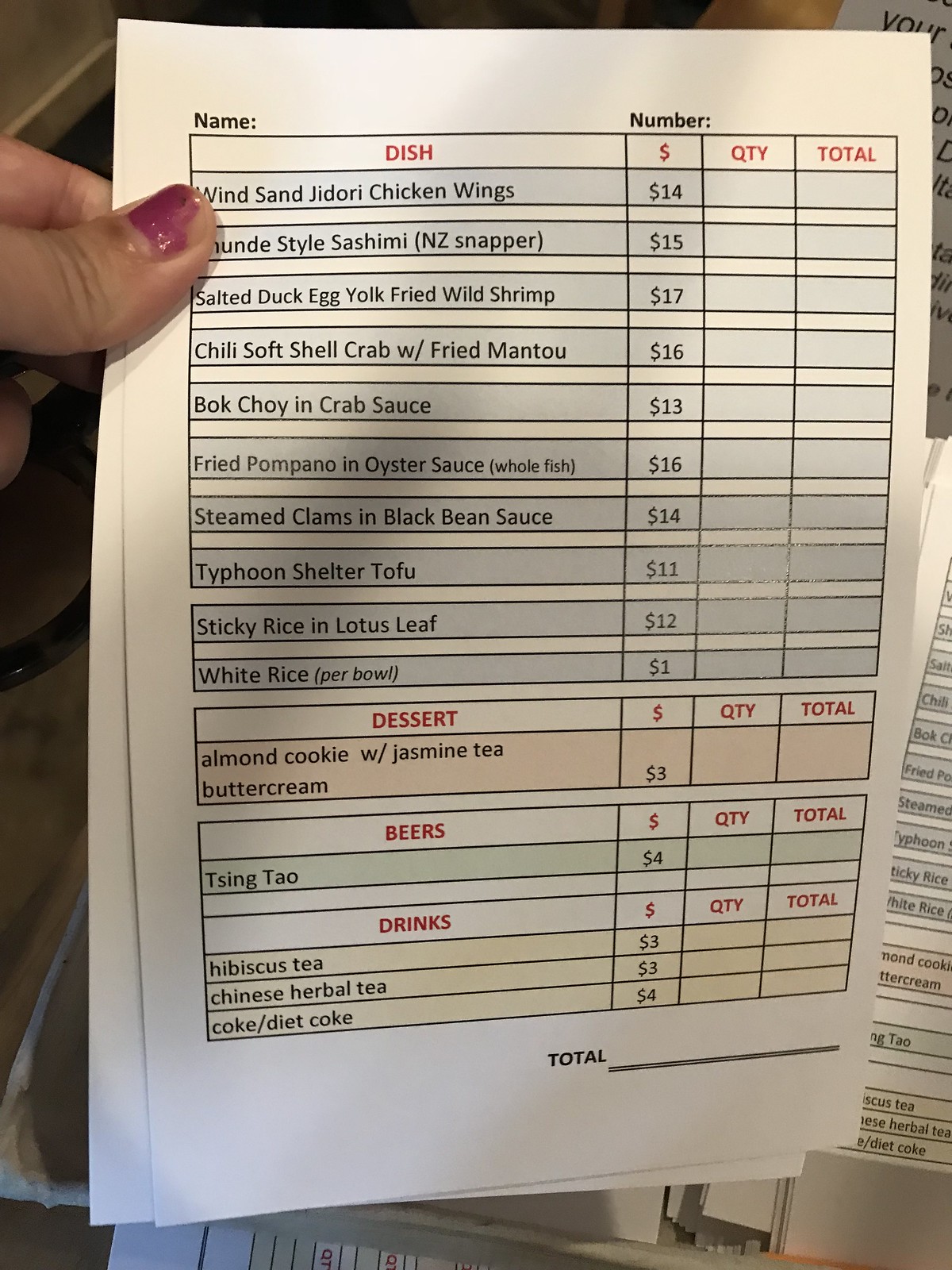In this vibrant, color photograph, a woman's hand with neatly painted pink nails can be seen holding a menu printed on white paper. The menu lists various delectable dishes, desserts, beers, and drinks, each with its respective price and total quantity. Notably, the menu includes:

- **Win San Giodori Chicken Wings**: $14
- **Sashimi or New Zealand Snapper**: $15
- **Salted Duck Egg Yolk with Wild Shrimp**: $17
- **Chili Soft Shell Crab with Fried Mantou**: $16
- **Bok Choy and Crab Sauce**: $13
- **Fried Pepano in Oyster Sauce**: $16
- **Steamed Clams in Black Bean Sauce**: $14
- **Typhoon Shelter Tofu**: $11
- **Sticky Rice in Lotus Leaf**: $12
- **White Rice, Purple**: $1

For desserts, the menu offers:
- **Almond Cookie with Jasmine Tea Buttercream**: $3

Under the beverages section, the options are:
- **Beer (Xingtao)**: $4
- **Drinks (Hibiscus Tea or Chinese Herbal Tea)**: $3
- **Coke, Diet Coke**: $4

The meticulous detailing and layout of the menu invite diners to indulge in a sumptuous variety of Asian-inspired culinary delights, promising a memorable dining experience.